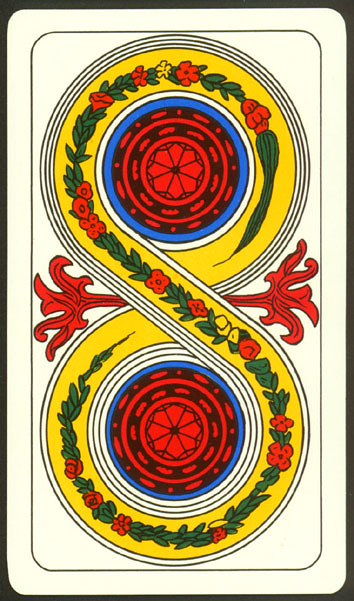The image depicts a meticulously designed piece of art, potentially a printed card or illustration, characterized by its vertical rectangular shape with rounded edges. The background is a soft light beige or ivory, bordered by a black outline, enhancing its print-like quality. Central to the design is an infinity shape—or a figure-eight—formed by two interconnected yellow circles. This yellow band is adorned with a continuous floral pattern featuring vibrant green leaves and red and yellow flowers, creating a striking visual contrast.

Within the top and bottom loops of the figure-eight, there are detailed red patterns with a central floral motif, reminiscent of a star with eight points, each divided into triangles. These intricate designs are encircled by white and blue outlines, adding layers to the visual depth. Additionally, a red horizontal bar connects the two circles at their midpoint, extending into flourishing floral shapes on either side, anchored by red stems. The overall composition suggests a blend of natural and geometric beauty, capturing the essence of a delicate, detailed artwork suitable for a decorative card.